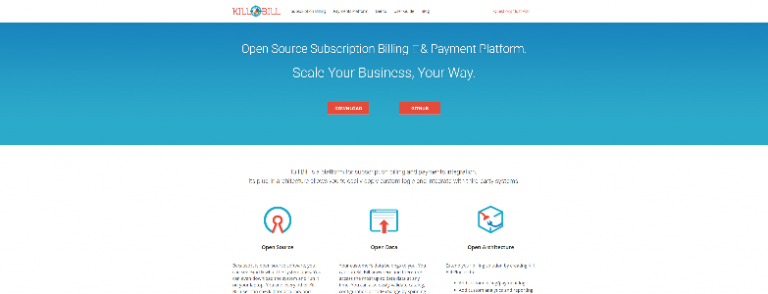The image appears to be a screenshot of a website called "Kill Bill," though it is of low quality, making finer text difficult to discern. The screenshot is notably wide, with much empty space on the left and right sides of the content. At the top, there is a horizontal menu bar featuring black text on a white background. Situated on the right side of this menu bar, there seems to be a "Sign In" or "Log In" option highlighted in red font.

Below the menu bar, there is a prominent blue rectangular banner that reads, "Open Source Subscription Billing and Payment Platform. Scale Your Business Your Way." Directly beneath this banner are two red rectangular buttons, likely serving functions such as "New User" or "Sign In."

Further down, the screenshot reveals black text alongside several icons: a lock icon, a file icon, and a cube icon with red and blue plugs appearing ready to connect. This section is presented on a white background.